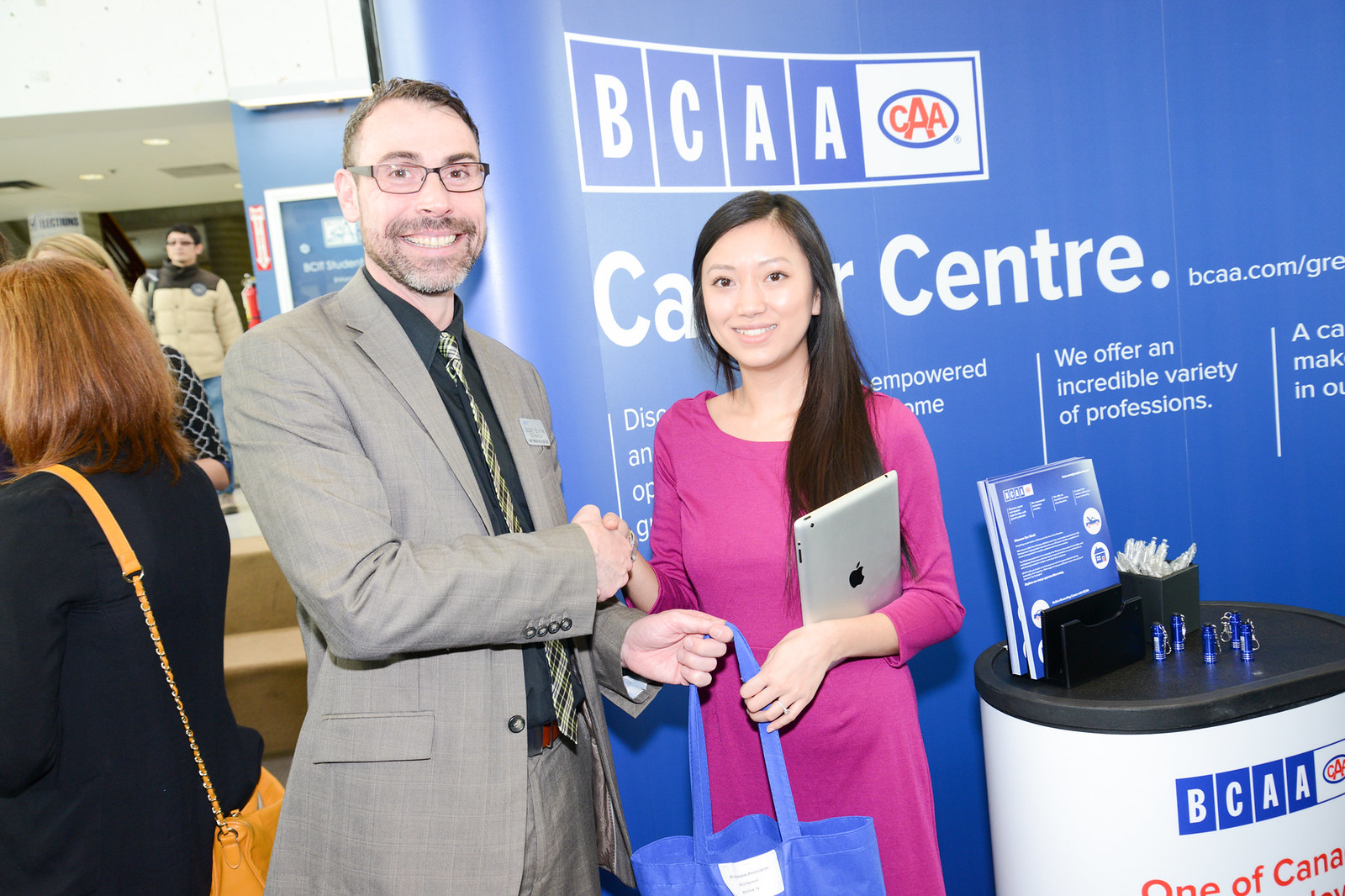The photograph captures a moment at the BCAA conference where a man and a woman are shaking hands in front of a booth marked "BCAA Center." The Asian woman, dressed in a pink dress, holds an iPad in her left arm and is receiving a blue gift bag from the man. She has black hair down to her chest and wears a wedding ring. The man, dressed in a gray suit with a dark blue undershirt, tie, and name tag, has glasses, a short gray beard and mustache, and short dark gray hair. Behind them, a sign reads "At BCAA.com, we offer an incredible variety of professions." Other attendees can be seen in the background, engaged in conversation, highlighting the busy atmosphere of the conference center.